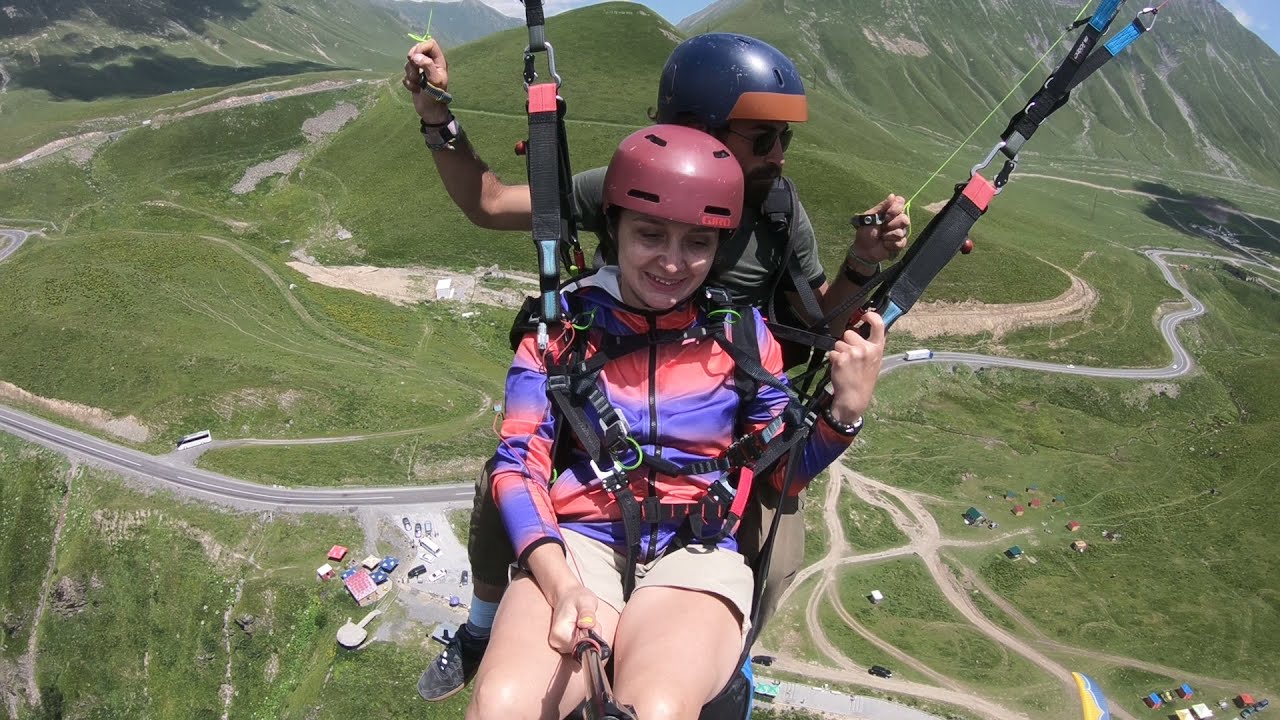This vivid selfie captures a thrilling moment of paragliding with a young woman and a man suspended in mid-air. The woman, prominently featured in the foreground, is wearing a red helmet and a red and purple jacket with a hood, paired with tan shorts. With a black selfie stick in her right hand, she snaps the photo that documents their adventure. Straps from the parachute are visibly hanging from her shoulders, securing her in place. Behind her, the man, identifiable by his blue helmet with orange trim and black sunglasses, skillfully maneuvers the bright yellow wires that control their descent. Below them, a green valley stretches out, intersected by an asphalt road and dotted with small houses. Towering in the distant background is a majestic mountain, completing the breathtaking scene.